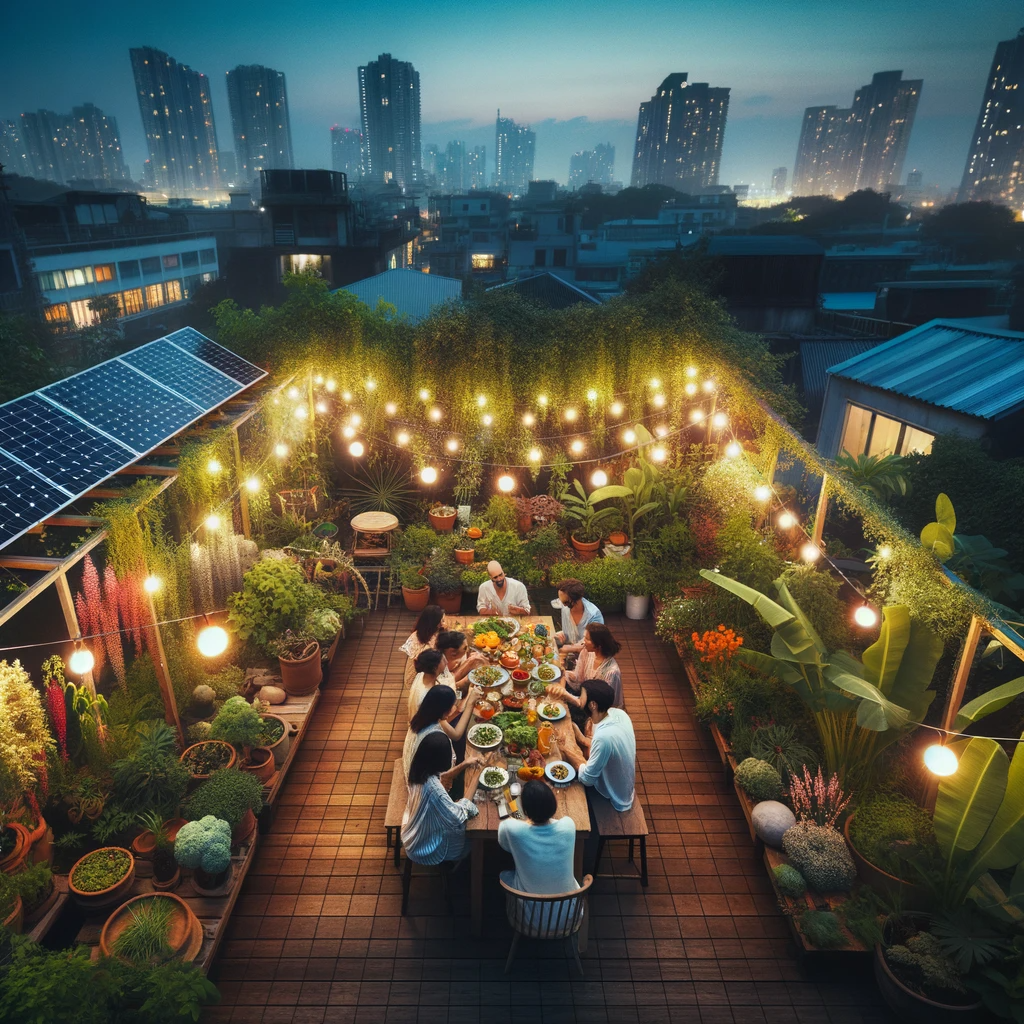The image captures an aerial view of a family gathered around a long rectangular table, enjoying a meal in a beautifully cultivated backyard garden. The table is flanked by two benches and a chair at each end, with a total of nine people seated: a male figure at the head of the table, a female figure at the opposite end, four people on one side, and three on the other. The ground beneath is tiled in a brown hue, adding a warm tone to the setting. They are surrounded by a vibrant garden featuring an array of green, red, and pink plants, contributing to the serene atmosphere.

Hanging above and behind them, soft whitish-yellow string lights illuminate the scene, while solar panels are visible to the left, hinting at a sustainable touch. In the far distance, the urban skyline is visible, suggesting this lush garden oasis is set within a residential area not far from downtown. The scene is detailed and visually rich, emphasizing the contrast between the tranquil garden and the bustling city skyline. Notably, the image appears to extend beyond traditional photography, exhibiting characteristics of graphic design or computer-generated realism.